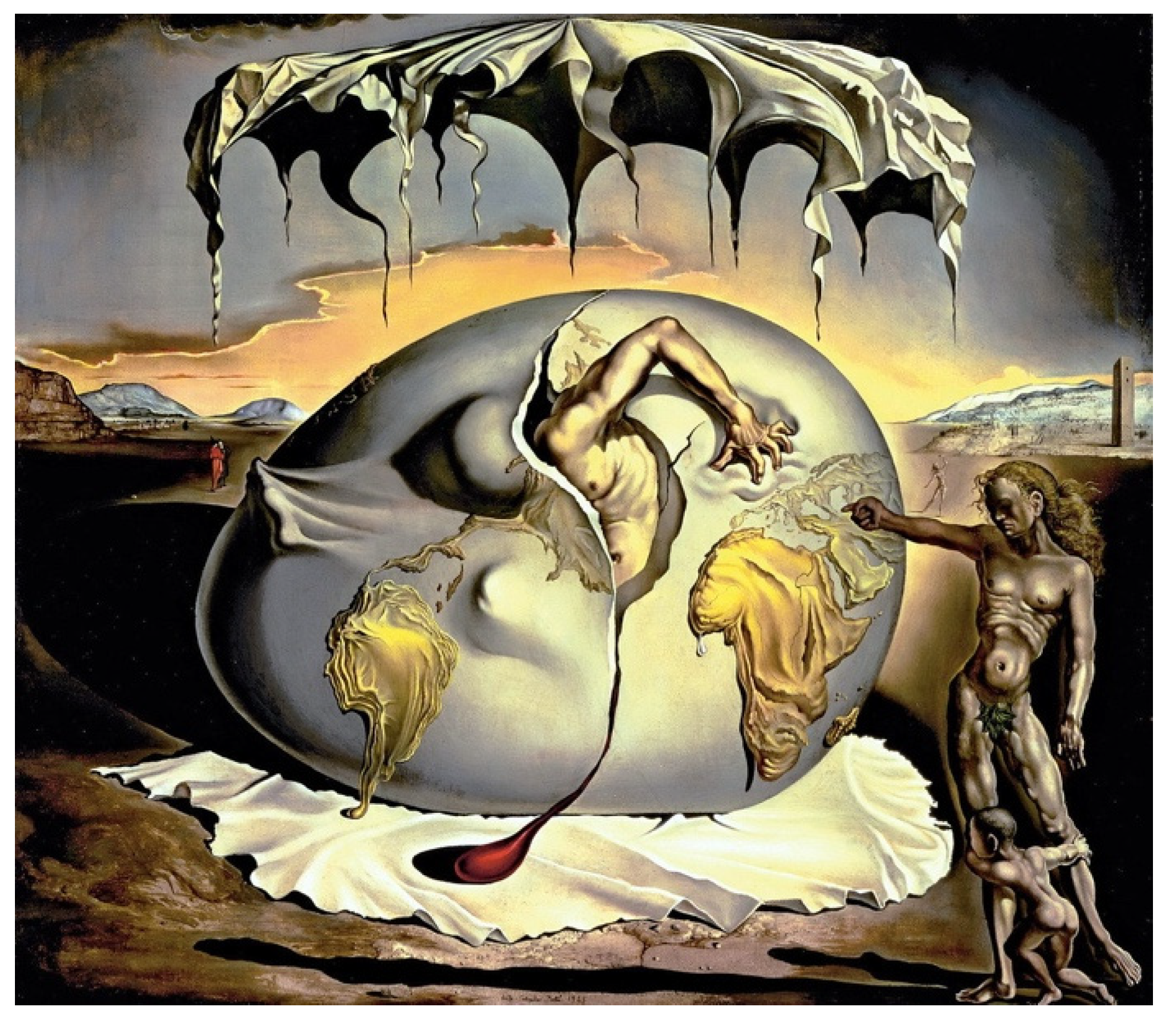The painting, reminiscent of Salvador Dali's surrealist style, is a somewhat eerie and detailed composition primarily rendered in tones of gray, yellow, red, white, black, and metallic tan. At the top center of the image, there is an unsettling, decaying piece of flesh shaped like an umbrella with spines hanging down the sides. The central focus is a large, rubbery, asymmetrical egg or distorted globe, pale and cracked down the center. Emerging from the interior of this egg or globe is a grotesque, unclothed man, with his torso and left arm protruding while his head is still partially inside.

This egg or globe rests on a white sheet or rag beneath it. To the right stands a bronze-colored, nude adult figure, possibly resembling an exoskeleton or a sculptural form, with long hair. This figure points towards the emerging man. At the base of their legs, a nude child clings, one arm wrapped around each knee, peeking towards the man attempting to break free from the egg. The entire scene conveys a surreal and almost melting appearance, filled with complex and haunting details that heighten its eerie atmosphere.